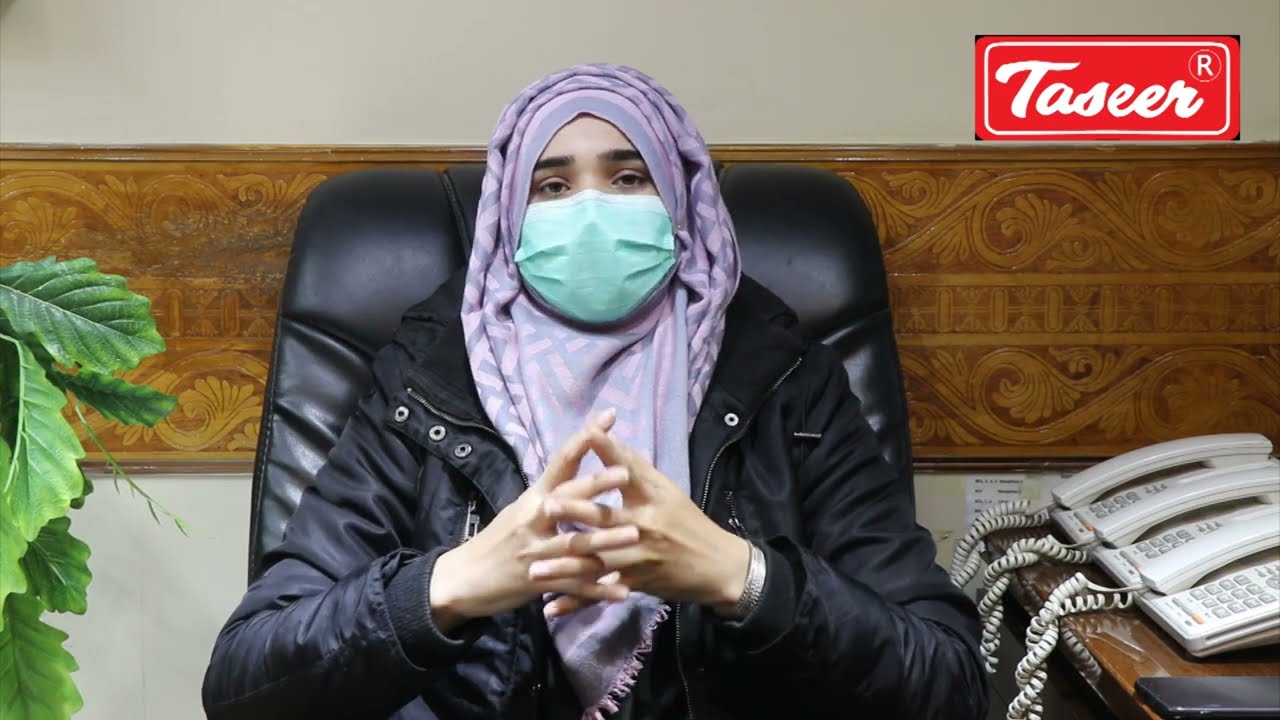In this indoor setting, which appears to be either an office or a home office, sits a Middle Eastern woman at the center of an image, addressing an unseen audience as if on a live stream or video call. She is comfortably seated in a tall black leather chair, dressed in a black jacket adorned with numerous buttons and snaps. Over her head, she wears a purple scarf or burka that drapes elegantly to the middle of her chest. Her face is partially obscured by a light blue surgical mask. 

Her hands, with fingers crossed but not clasped, rest in her lap. To her right, a shiny wooden desk holds a row of three white corded telephones. In the upper right corner of the image, the word "TASEER" (T-A-S-E-E-R) is prominently displayed in a red bar with a white border. 

Off to the left side of the image, a green plant adds a touch of life to the scene. The color palette of the image includes off-white, red, white, purple, light blue, tan, black, green, and gray, creating a composed and detailed environment.